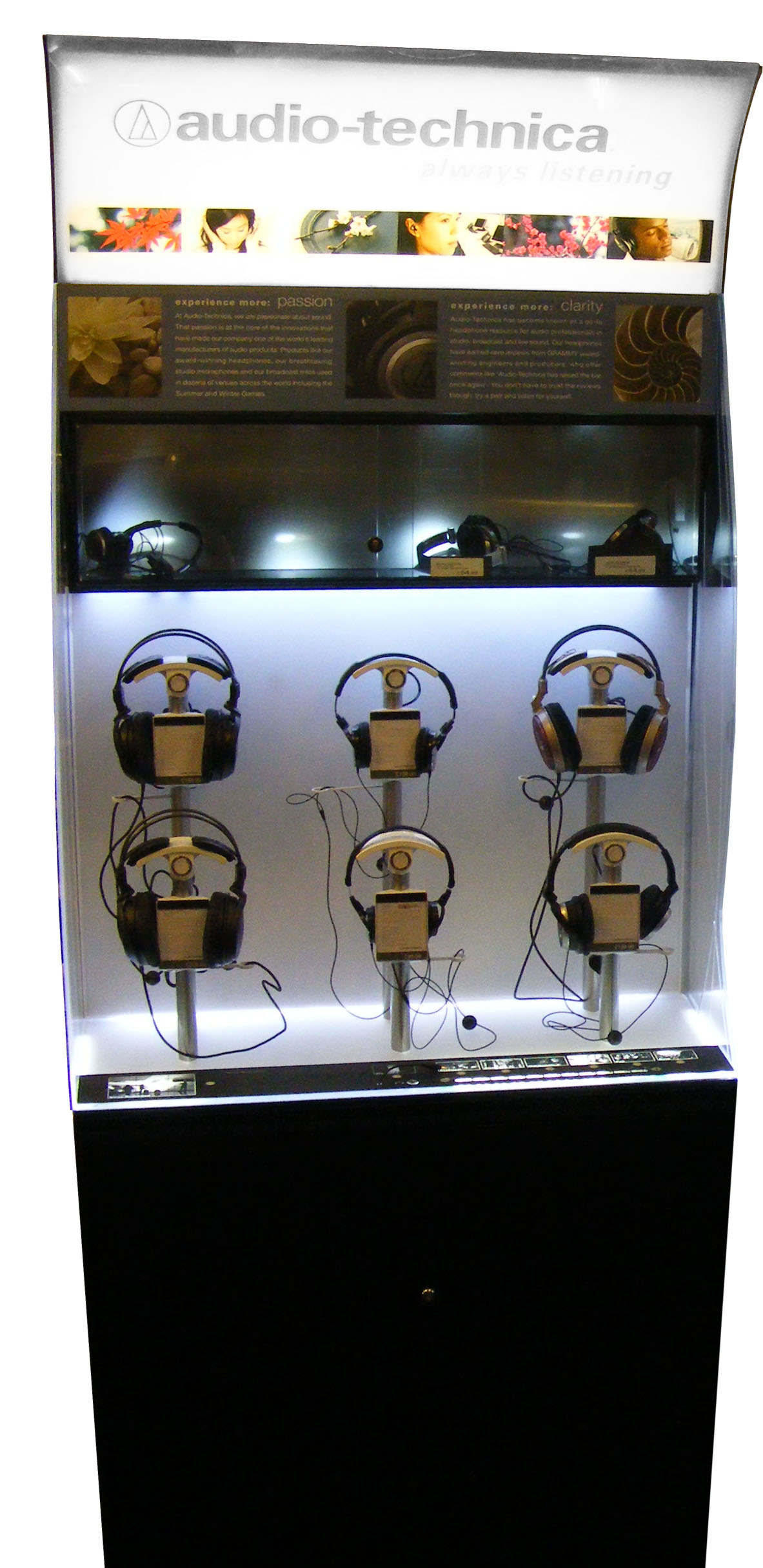The image shows a vertical, rectangular kiosk designed to resemble an old-school arcade console and it prominently features Audio-Technica branding at the top in gray lowercase letters on an illuminated white background. The central section of the kiosk displays six pairs of headphones arranged in two rows of three. Each row consists of individual stands—some viewers describe these stands as raising the headphones to eye level. Beside the main display, there are also images of people using the headphones, adding context and appeal to the setup. The headphones themselves are black and gold, with varying sizes of earpieces. They're connected via cords, allowing potential users to listen to preset audio samples to test the quality. The elegant display invites users to interact with the headphones while highlighting the premium design and audio experience from Audio-Technica.